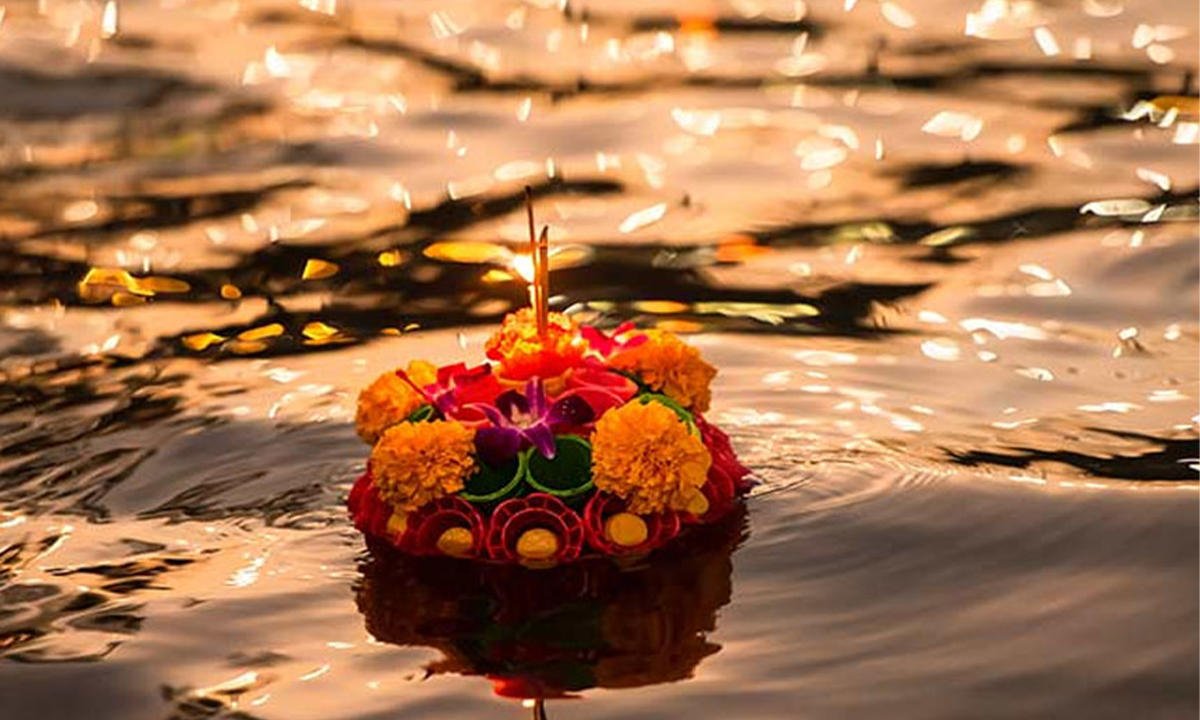This image captures a vibrant floating flower arrangement on a body of water. At the heart of the arrangement are vivid yellow carnations, surrounded by smaller, round structures in hues of red, green, and purple. These are intricately bunched together, creating a visually stunning display. The water beneath them appears grayish-black or coppery and is alive with ripples and reflections, including golden and white splotches caused by sunlight. The overall setting is undoubtedly outdoors, with the sun shining down, adding a dynamic interplay of light and shadow on the water surface, enhancing the beauty of the floating arrangement.